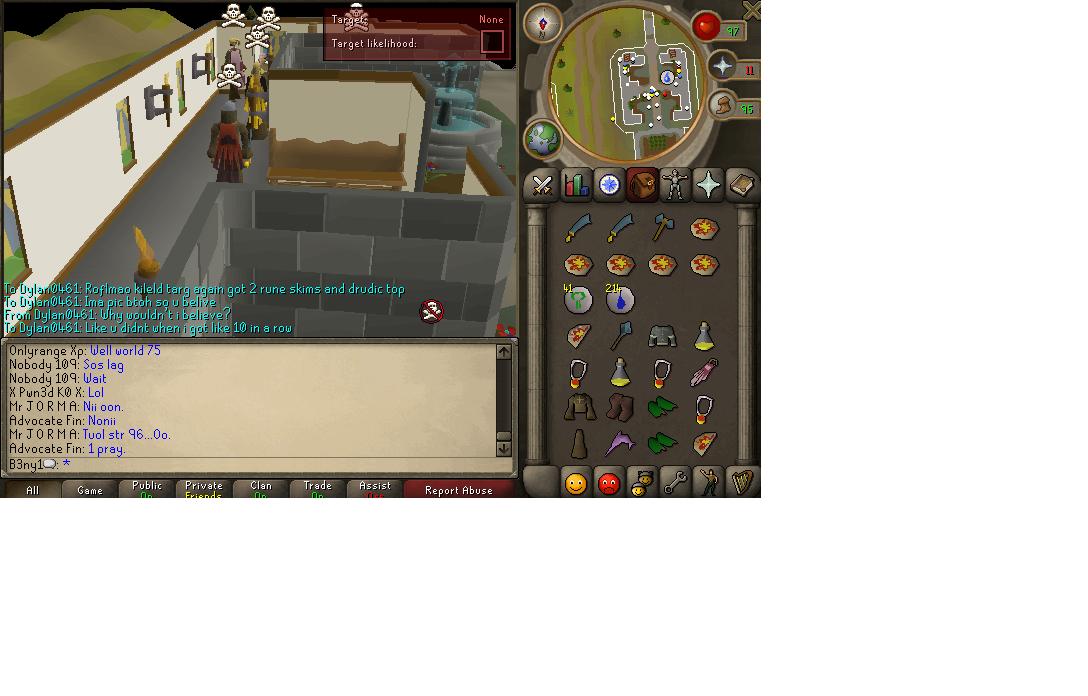The image depicts an early CGI-style computer game with a distinct, blocky animation style reminiscent of older, less modern graphics. The main section of the screenshot showcases the gameplay action, where a knight character stands inside a castle-like hall with gray stone walls, windows displaying an outside view, and torches casting an orange glow. Above this scene, a banner reads "Target: none, Target likelihood," beside which several skulls with crossed bones are displayed, possibly indicating a target marker system.

To the right, there is a detailed game map in the top corner, displaying various icons and colored dots (yellow, blue, red, and white) representing different elements of the game world, including a gray shape highlighting the player’s current building. Below this map, the player's inventory is visible, containing items such as swords, axes, necklaces, and clothing.

At the bottom of the screen, a beige chat window with black and blue text shows player communications. The overall immersive atmosphere is enhanced by the intricate stonework, scattered medieval-themed objects like skulls, skeleton pirates, and banners, creating a vivid medieval fantasy setting.